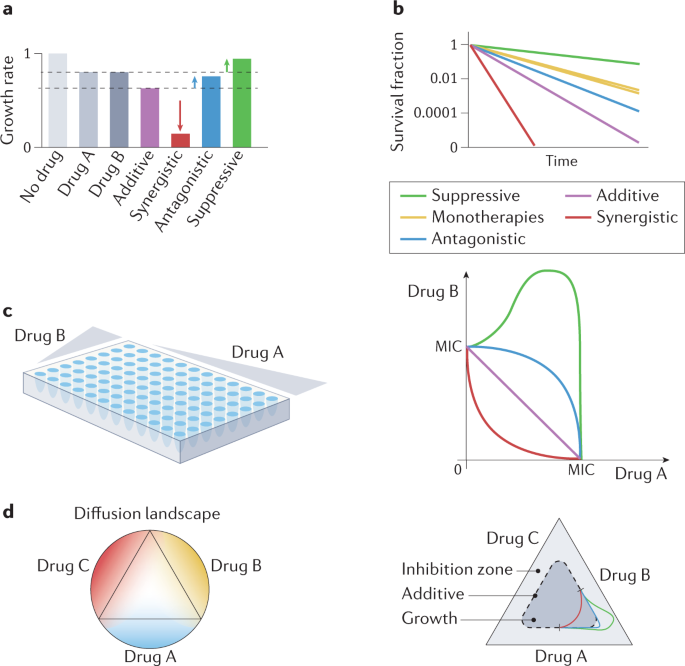The image displays a series of six scientifically detailed graphs on a plain white background, all related to pharmaceutical analysis. Each graph is labeled from A to F, and they measure various pharmacologic parameters.

- **Graph A (Upper left)**: A bar graph indicating growth rate, ranging from 0 to 1 on the y-axis, comparing "No drug," "Drug A," "Drug B," "Additive," "Synergistic," and "Antagonistic" effects. Synergistic interactions show a significant decrease indicated by a downward arrow, while antagonistic and suppressive interactions show increases with upward arrows.

- **Graph B (Upper right)**: A line graph that maps the survival fraction, ranging from 0 to 1, against time. It features five different colored lines that begin at the survival fraction of 1 and descend over time, demonstrating various drug effects on survival rates.

- **Graph C (Middle left)**: Depicts a comparison between "Drug A" and "Drug B" using a scatter plot of blue dots contained within a case. This graph possibly highlights differences in response or efficacy between the two drugs.

- **Graph D (Middle right)**: Another bar graph emphasizing Minimum Inhibitory Concentrations (MIC) of "Drug B" labeled on the y-axis, with values compared to "MIC and Drug A" on the x-axis, from 0 onwards.

- **Graph E (Lower left)**: A diffusion landscape graph, illustrating drug interactions within a circular layout where a triangle is inscribed. The circle is color-coded into sections of yellow, red, and blue to indicate specific regions associated with "Drug A," "Drug B," and "Drug C."

- **Graph F (Lower right)**: Shows an intricate diagram featuring a larger triangle with a smaller triangle inside it, labeled "Inhibition Zone," "Additive," and "Growth." Edges of the triangle are marked with "Drug C," "Drug B," and "Drug A," indicating comparative diffusion or inhibition zones among the three drugs.

This comprehensive layout evidently provides an in-depth comparison of several pharmaceutical indicators, focusing on growth rates, survival fractions, MIC values, and drug diffusion landscapes.